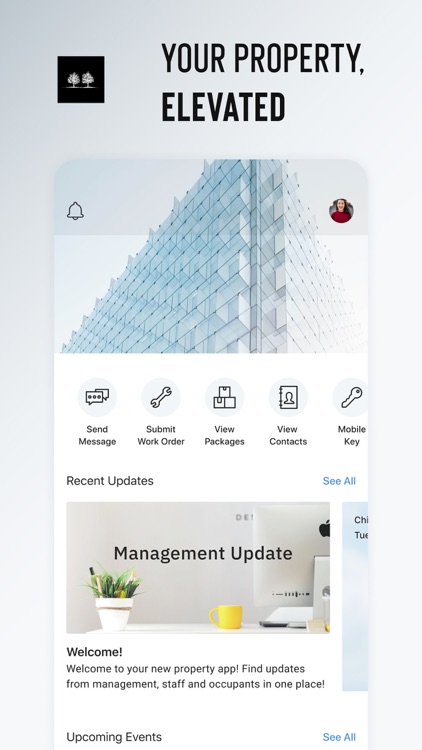This detailed caption explains the contents of the image:

The image features a screenshot set against a light gray background. At the top, prominent black text reads "Your property elevated." In the upper left corner, there is a black square containing two white, illustrated trees. Below this text, there is a digitally-rendered image of an apartment building composed of mini cubes.

In the upper right corner of the gray box, a circular photograph shows a female. Below, a series of black text labels are arranged horizontally, reading from left to right: "Send message," "Submit work order" (accompanied by an icon of a wrench), "View packages" (with an illustration of three boxes), "View contacts," and "Mobile key."

The lower portion of the image displays a photo containing a white potted plant, a yellow mug, and part of a laptop with an Apple logo on its back. Overlaying this photo, bold text states "Management Update," followed by the message "Welcome to your new property app."